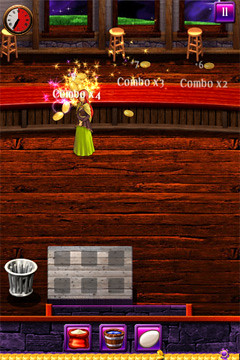This screenshot appears to be from a vintage video game, likely originating from the 1980s or 1990s, depicting a bar scene. The setting features a hardwood floor and a bar in the background, distinguished by a reddish wooden countertop. At the bar, a woman with red hair is present, dressed in a brown blouse and a green dress. Gold coins are animated, flying around her, accompanied by white text displaying "Combo X4," "Combo X3," and "Combo X2." In the top left corner of the screen, a clock is visible, adding another layer of detail to this nostalgic game snapshot.